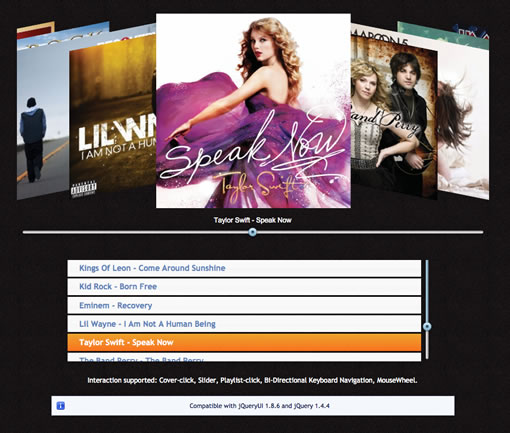This image captures the main interface of a music website, showcasing a sleek, modern design with a predominantly black background. The upper half of the page prominently displays a selection of album covers, artist names, and album titles. 

Starting from the left, the first album cover displays the back of a person walking down a long road, dressed in dark clothes with only the back of their head visible. Next to it is another album cover that features what appears to be a detailed, textured ground with black and brown walls and partially visible gold accents. The text on this cover reads "little w..." and "I am not a HU..." but both are notably cut off.

In the center of the album lineup, a full cover of Taylor Swift's album "Speak Now" stands out. Taylor Swift is pictured with wavy hair, looking directly at the camera while wearing a purple dress, her left arm extended in front of her. The album title is written in cursive, and "Taylor Swift" is displayed in gold below it.

To the right, another album cover shows a woman with short blonde hair and pale skin, dressed in a white crop top with her hands on her hips. Only her left arm is visible as the right side of the cover is partially obscured by the Taylor Swift album.

Further to the right, there's an image of a person with shoulder-length brown hair, pale skin, holding a round guitar, and dressed in a blue suit. The furthest right album is only partially visible, showing a white background with a bed and a woman's brown hair blowing in the wind, with "Maroon 5" faintly visible at the top.

Below this display is a horizontal line, beneath which the title "Taylor Swift - Speak Now" is prominently highlighted. A circular button featuring a black house icon is centrally placed below this.

Further down, a list of other artists and their albums is presented in blue text:
- **Kings of Leon** - "Come Around Sundown"
- **Kid Rock** - "Born Free"
- **Eminem** - "Recovery"
- **Lil Wayne** - "I Am Not a Human Being"

At the bottom of this list, in an orange-highlighted bar, is another mention of "Taylor Swift - Speak Now," in white text.

A note at the bottom, also in white text, mentions various functions supported by the website, including "interaction supported, cover click, slider, playlist click, bi-directional keyboard navigation, and mouse wheel."

Finally, a horizontal information bar runs across the bottom of the page, featuring a blue box on the left that states "compatible with Query UI 1.8.6 and jQuery 1.4.4."